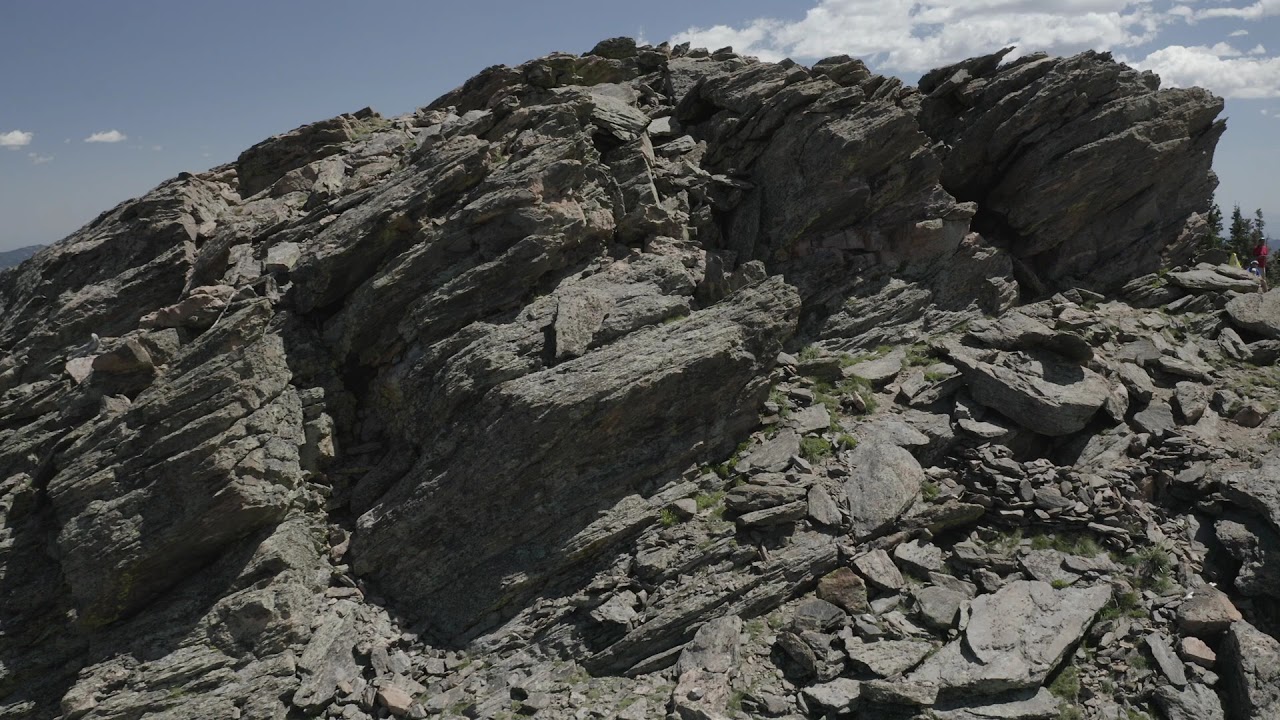The photograph captures the rugged face of a rocky mountain, characterized by its unusual, jagged formations that create a slate-like appearance. These rock structures, which seem to blend uniformly into one another, are slanted at an approximate 30-degree angle, giving the impression of layered stacks that look like they are peering up towards the sky. The image reveals a chaotic assortment of loose rocks breaking off and cascading down the mountain, with slivers and chunks of rock scattered everywhere. Despite the overwhelming rocky surface, sporadic patches of grass and greenery can be spotted amongst the debris. Towards the top left and right corners of the picture, a blue-gray sky with fluffy white clouds is visible. On the very far right side of the image, a small figure wearing a red shirt and white hat stands out against the rocky backdrop, gazing at the camera from a distance, adding a touch of humanity to the otherwise stark and barren scene.